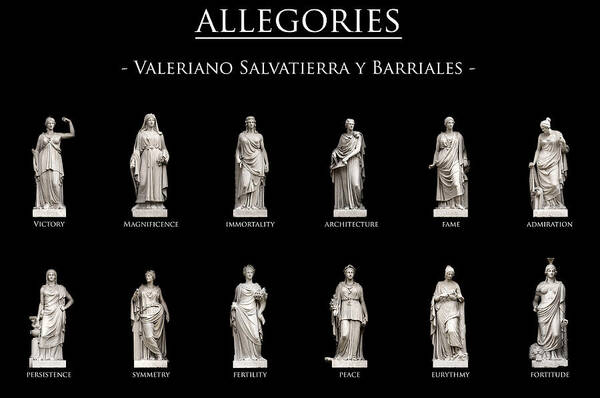The image features a black background with the title "Allegories" in off-white, bone-white text at the top, underlined for emphasis. Directly below the title, in capital letters, it reads "- Valeriano Salvatierra y Borealis -". The image showcases two horizontal rows of statues, each with their respective titles beneath them. The top row includes: Victory, Magnificence, Immortality, Architecture, Fame, and Admiration. The bottom row features: Persistence, Symmetry, Fertility, Peace, Urithmy, and Fortitude. The statues, reminiscent of Roman or Greek deities, represent both gods and goddesses, encapsulating various virtues and abstract qualities.